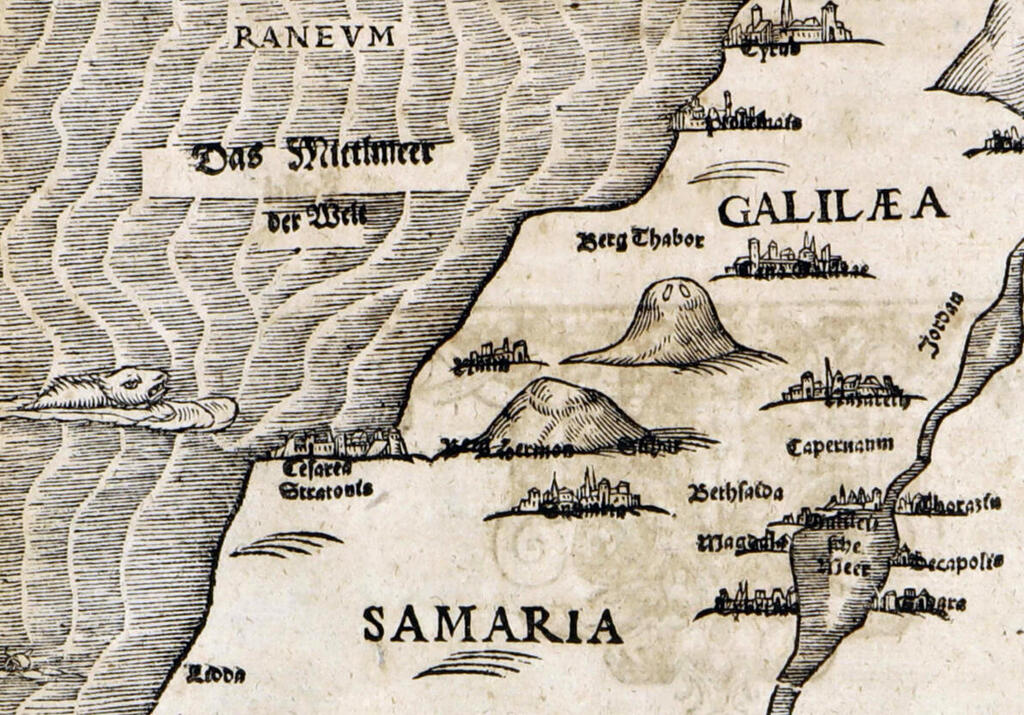This is a detailed black and white map illustration with a beige or off-white surface, depicting various regions and landmarks from the Middle East, possibly from biblical times. The largest text labels the regions of Samaria and Galilea, suggesting these as the central focus areas. To the left, there's an area resembling a body of water with waves, which includes the text "RONEVM" and a beaver-like creature swimming. There are several labeled buildings, including 'BERG HARBOR' and 'CAPRNUM,' indicating specific locations of interest. The Jordan River is depicted flowing through the map, alongside mounds resembling mountains or rounded hills. Some obscure and likely German text, such as "Das Miertmierger Wille," appears in the illustration, adding to the old-world charm of the map. This map provides a historical and geographical overview of significant areas, possibly tracing routes and locations pertinent during the time of Jesus.